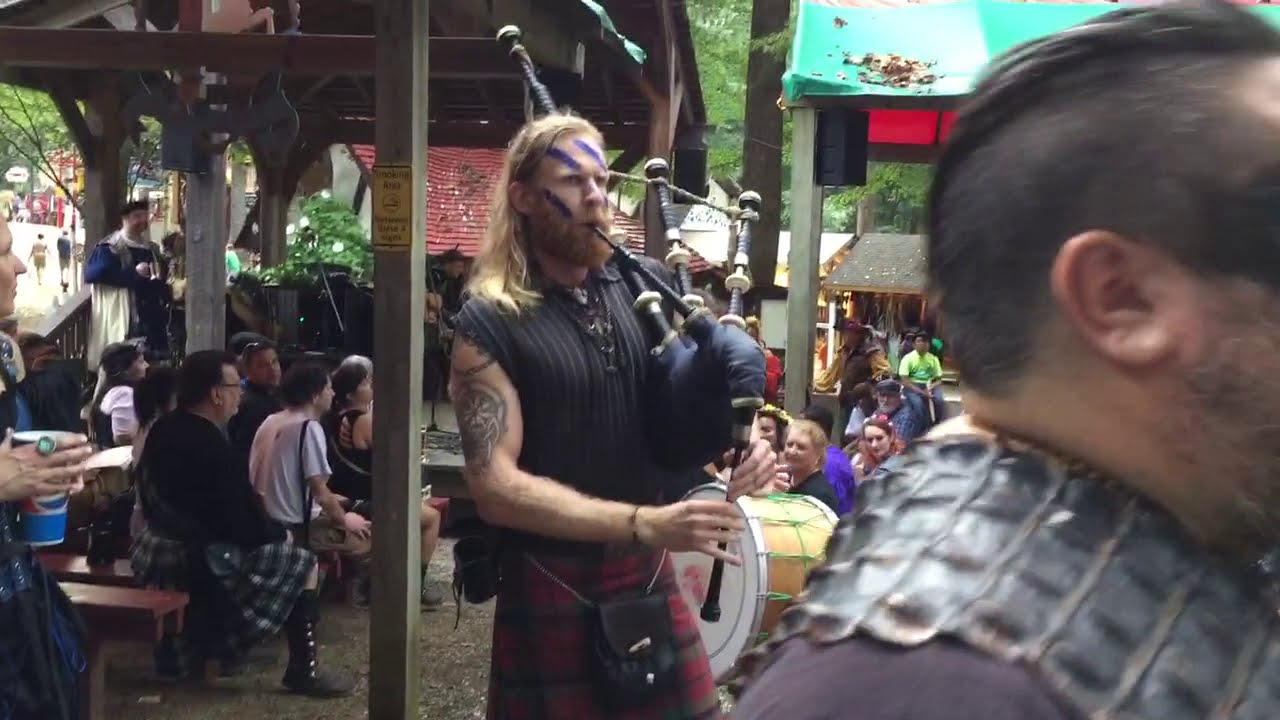This image captures a lively outdoor festival scene during the daytime. Central to the photograph is a young man of Caucasian descent, adorned in a red and black kilt with a purse hanging in front. He stands out with his full red beard and shoulder-length blonde hair, and his face is strikingly decorated with three purple diagonal stripes. He is absorbed in playing the bagpipes, holding the instrument predominantly in his left hand, with his right hand, which sports a bracelet, manipulating the stem. A notable feature is a circular tattoo with a tribal design on his right bicep.

Behind him, slightly to the right, is a large bass drum. The right side of the image is partially occupied by another man who is very close to the viewer, sporting dark brown hair that is shaved on the sides with a small mohawk. He wears an armor vest over a dark mauve shirt and has black paint around his temples, contributing to the festive atmosphere. 

The setting is vibrant with numerous attendees dressed in kilts and Renaissance costumes, sitting on benches and tables, walking, or standing beneath wooden and material canopies to the left and right, respectively. The festival ambiance is further enriched by scattered performances and people watching in an open picnic area, indicating a jubilant Scottish or Renaissance theme.